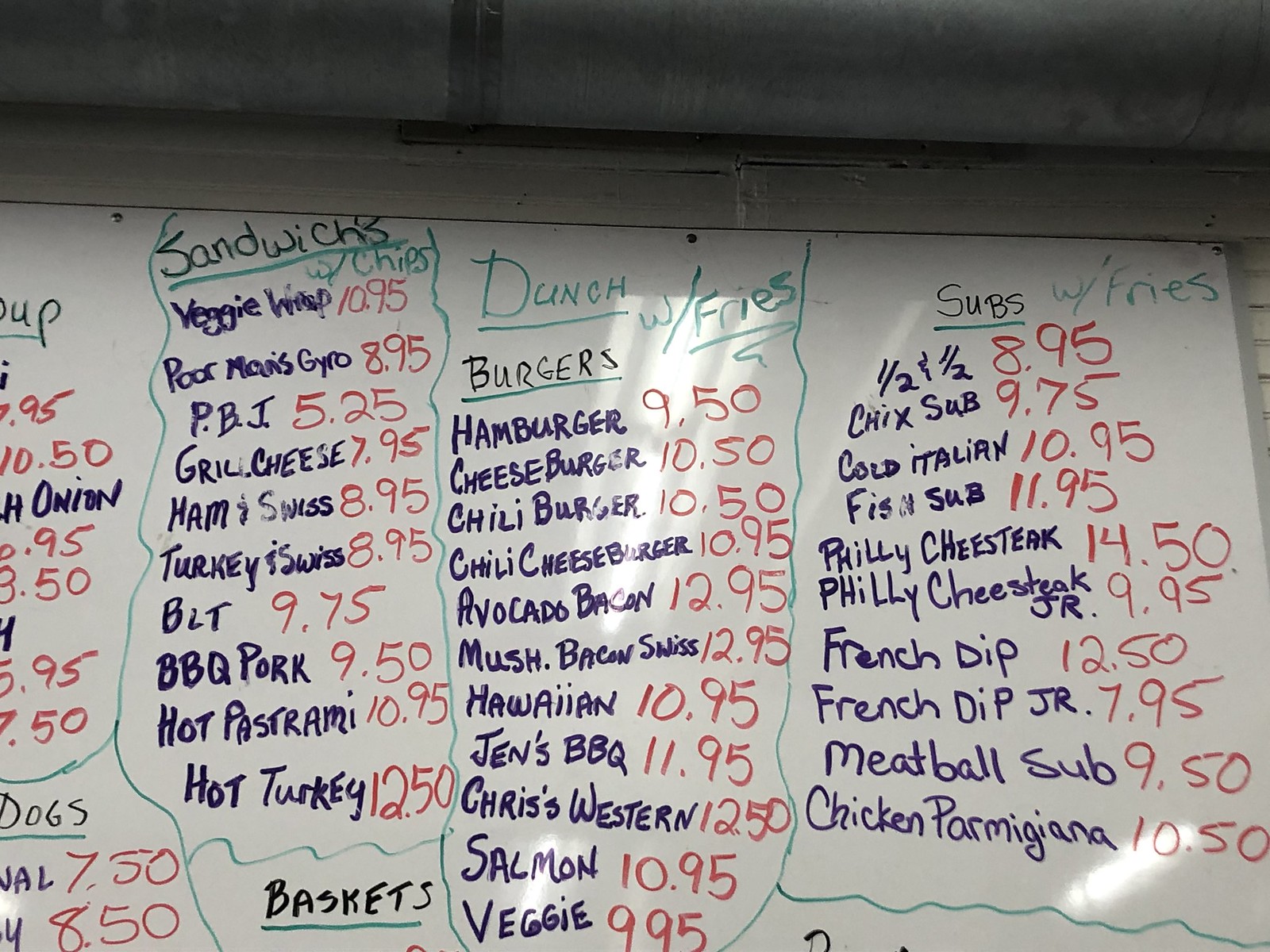A whiteboard menu divided into four columns listing various food items and their prices, with headings in green, food items in purple, and prices in red. The far-left column is partially cut off, making it hard to read fully, but it features sandwiches with chips. Examples include a BLT for $9.75, BBQ pork for $9.50, and a hot turkey sandwich for $12.50. The middle column is labeled "Dunch" – a blend of lunch and dinner – and offers burger options that come with fries, such as a hamburger for $9.50, a cheeseburger for $10.50, and a salmon burger for $10.95. The far-right column lists subs with fries, including a cold Italian sub for $10.95 and a fish sub for $11.95.